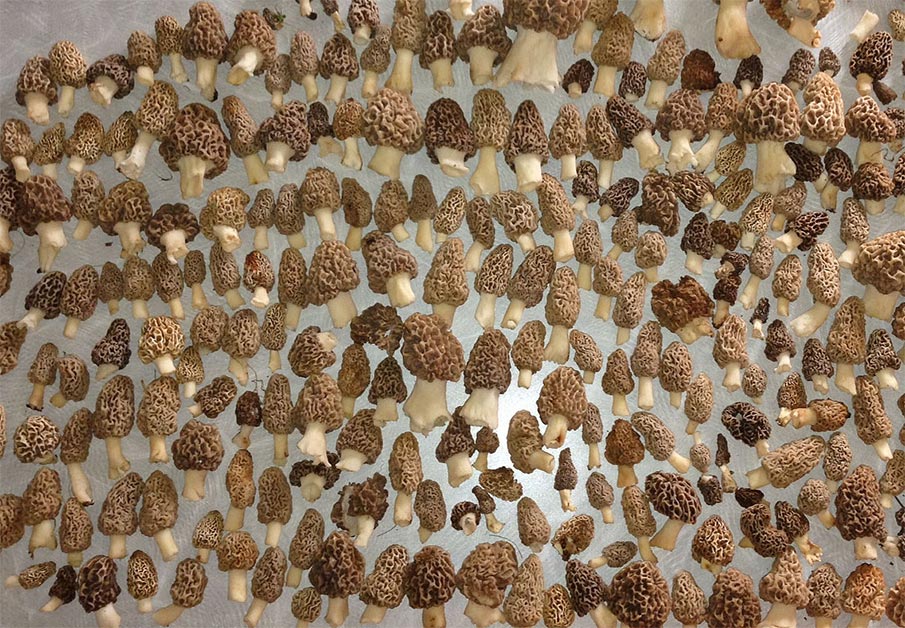The image showcases a large assortment of mushrooms arranged on a gray, possibly fabric-covered surface, as though they are being dried. Featuring varying sizes and colors, the mushrooms primarily exhibit tops that resemble sponges, ranging from tan and reddish-brown to darker brown hues. Most stems are cream to white shades and appear truncated. The mushrooms are uniformly laid out in a single layer without overlapping. Notably, smaller tan mushrooms are grouped together on the left side, while larger, darker brown mushrooms dominate the center. Some mushrooms exhibit bullet or arrowhead shapes, adding to the diversity of their presentation. The detailed arrangement and varied characteristics make it unclear whether the mushrooms are real or perhaps crafted from materials like plastic or clay.